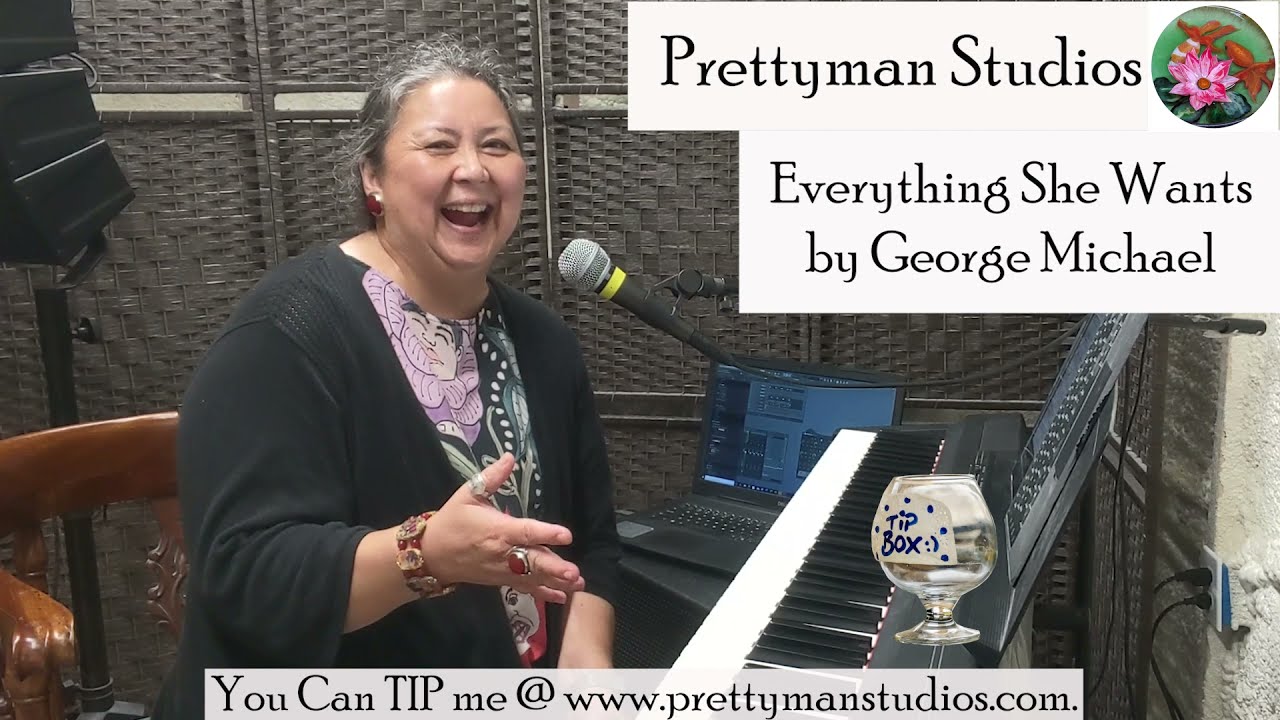The image features an older woman with a touch of gray in her hair, seated in front of a keyboard with a microphone positioned in front of her and a laptop with audio software open to her left. She is adorned in a long black over-shirt with a black floral-patterned shirt underneath, displaying purple flower petals near her neck. The woman is captured mid-laugh, her mouth open and her right side facing the camera, as she sits in a brown wooden chair. To the right of the woman, a white rectangular banner reads "Pretty Man Studios" accompanied by a circular logo featuring a pink flower and two koi fish—one orange and one orange and white striped. Below this, another white rectangle includes the text "Everything She Wants by George Michael." Additionally, at the very bottom of the image, there is a slightly off-white rectangle with black text that says, "You can tip me at www.prettymanstudios.com." The right side of the keyboard along with a fishbowl acting as a tip container are also visible. The setting is a small room with a basket weave wall to the left.